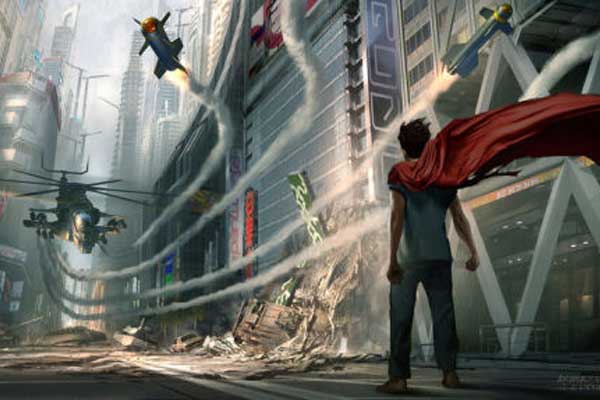In this dynamic and intricately detailed digital artwork, a young man stands resolutely on the right side of the image, set against a backdrop of a cityscape in turmoil. He is wearing a light blue, short-sleeved t-shirt, dark blue pants, and simple flat shoes. His most striking feature is a large red cape that flows dramatically from his shoulders, extending toward the top right central part of the image. The young man, who has dark skin and bushy black hair, faces an imminent threat with fists clenched behind him, seemingly in a defiant stance. The background is a chaotic jumble of dark gray, silver, and white, with shattered buildings and towering city structures fragmenting into the sky. 

In the left portion of the scene, several dark gray airplanes leave curving trails of white smoke as they weave between the city towers. Flying low and aggressively into the scene is an attack helicopter, hovering just above the ground. Multiple missiles, leaving distinct smoke trails, streak towards the young man, creating an intense, action-packed atmosphere. The overall ambiance suggests a post-apocalyptic or futuristic setting, reminiscent of a scene from a high-stakes video game or movie. Despite the desolation, the presence of some illuminated buildings hints at lingering remnants of civilization, enhancing the depth and narrative complexity of the scene.